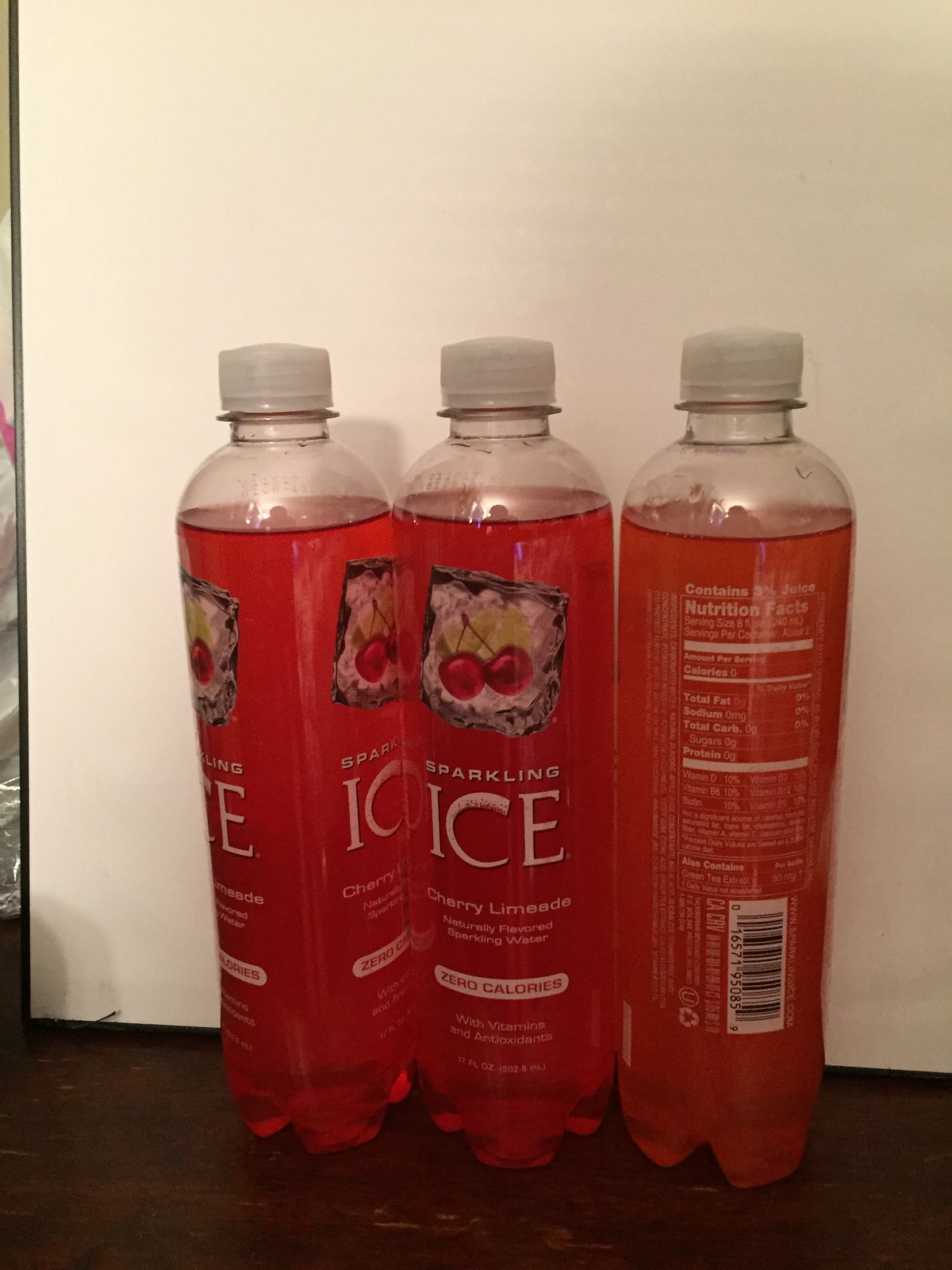The close-up image showcases three tall, slim plastic drink bottles, all containing the same beverage but with slight variations in color. Each bottle holds approximately 600 milliliters or 12 ounces. The bottles are topped with serrated plastic caps, and the liquid inside is a reddish-orange hue. Notably, the bottle on the far right features a more pronounced orange tint compared to the other two. 

The base of each bottle is not flat; instead, it has triangular-shaped, indented grooves providing stability. The front of the middle bottle is prominently displayed, showcasing a label with "Sparkling ICE" in bold white lettering, followed by "Cherry Limeade" in smaller text. It is indicated that the drink is naturally flavored sparkling water with zero calories and enriched with vitamins and antioxidants. The upper part of the label features a graphic of two cherries resting on a leaf against an icy backdrop.

We see the side of the left bottle and the back of the right bottle, which displays a nutritional table mainly filled with zero values, except for the vitamins and antioxidants content.